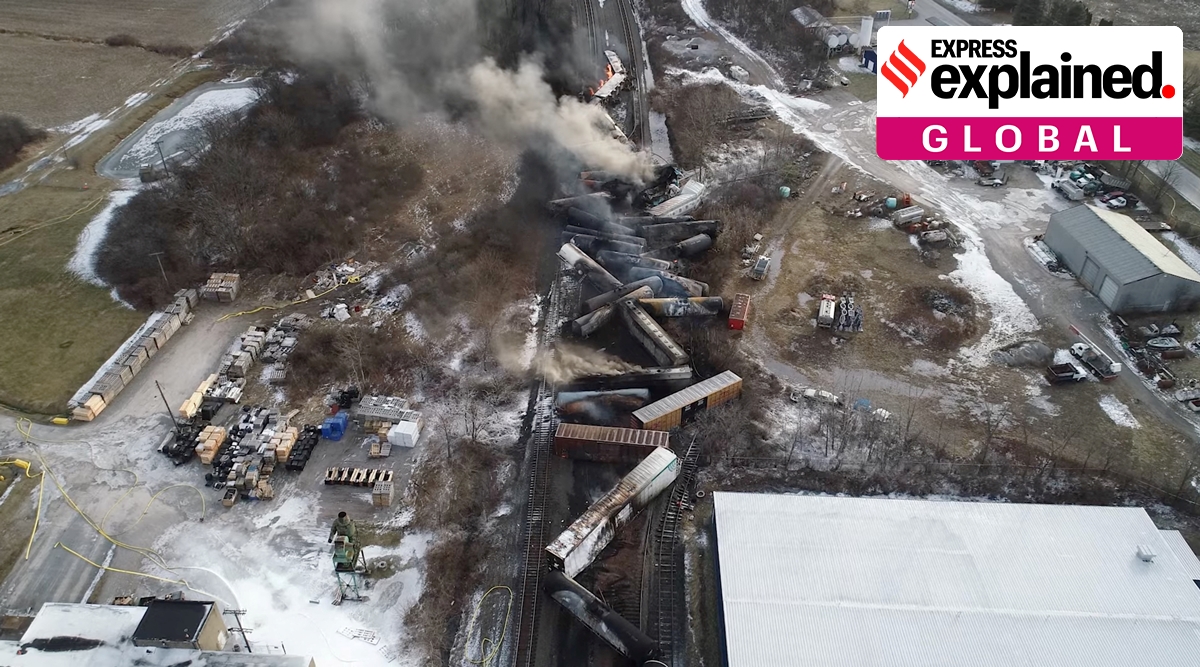This horizontally aligned rectangular aerial photograph vividly captures the aftermath of a catastrophic train derailment. Dominating the center of the image, chaos reigns with twisted, overturned train cars—tank cars, box cars, and hoppers—strewn in various directions amidst a landscape shrouded in thick, white and brown smoke, with flames visible in some areas. The smoke drifts towards the upper left, emphasizing the scale of the disaster. In the upper right corner, a distinctive graphic overlay features a white background with "EXPRESS EXPLAINED" in dark black text followed by a red period, and below it, "GLOBAL" in white letters on a pink background. The lower right of the photograph shows a flat-roofed, white building, part of an industrial area surrounding the wreck. Vehicles and possibly emergency response teams are scattered throughout the scene, and the area to the left includes roads, flat lands, and crops, starkly juxtaposed against the wreckage. Some vehicles and pallets are visible, indicating a mix of industrial and rural elements in the vicinity of this devastating derailment.